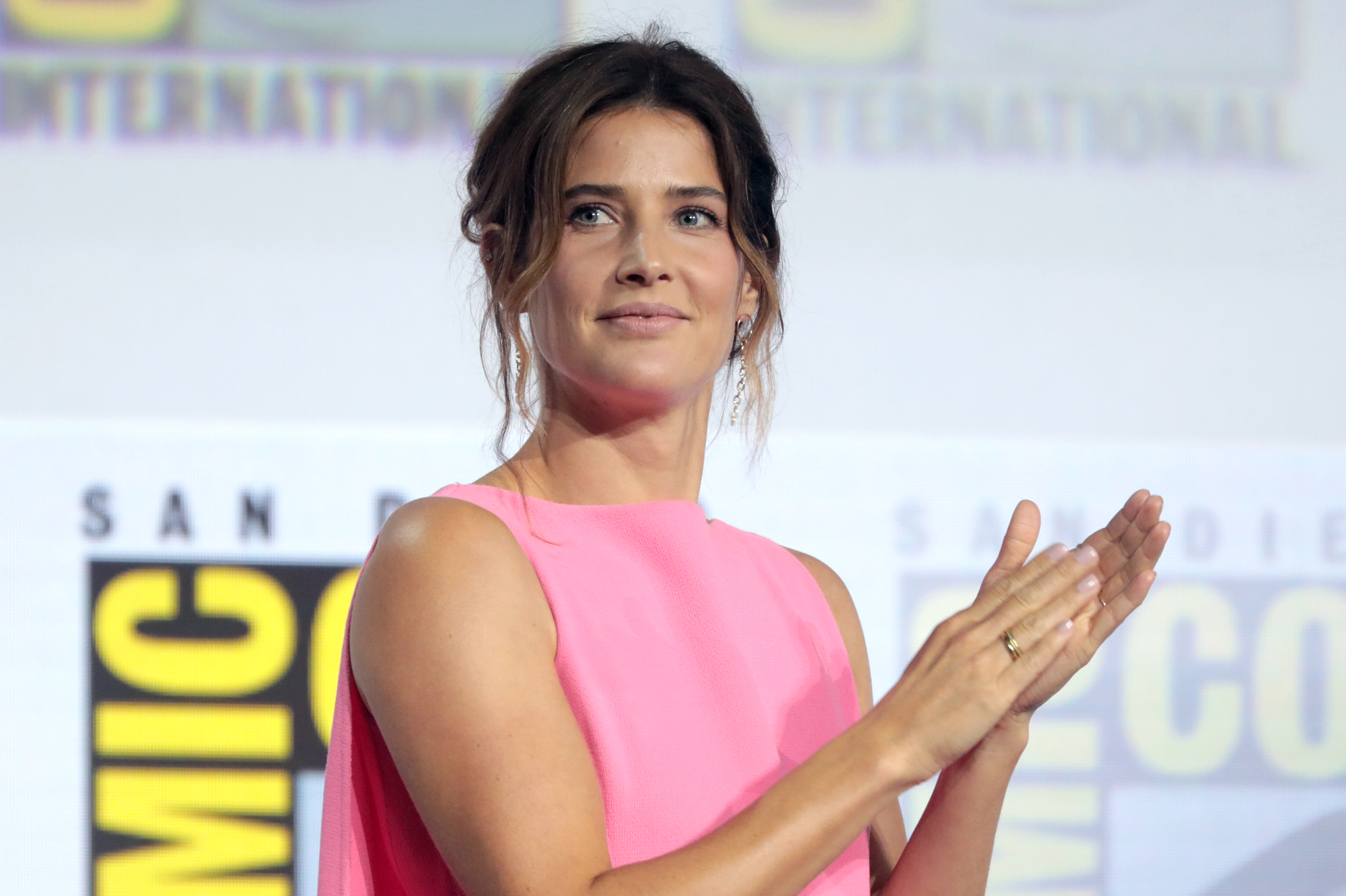In this photograph, a woman is standing in front of a white wall adorned with repeating San Diego Comic-Con logos. The logo features black text reading "San Diego" surrounding a square outline with yellow text inside that reads "Comic-Con." The woman is depicted from the upper stomach to the top of her head, looking towards the upper left side of the photo. She is dressed in a pink, sleeveless blouse and has neatly put back brown hair, gathered into a bun with lighter brown ends. Her complexion is clear and slightly shiny, suggesting well-maintained skin. She wears gold dangling earrings, a gold ring on her right ring finger, and understated makeup. Her nails are manicured, and she has green or blue eyes. The woman appears to be clapping or holding her hands together to the right of the frame, creating a pose that reveals the definition in her neck. The background, filled with text elements like "S-A-N" and "M-I-C," and colors such as pink, tan, yellow, white, light blue, and black, complements the composition, though the indoor or outdoor setting and the time of day are indeterminate.